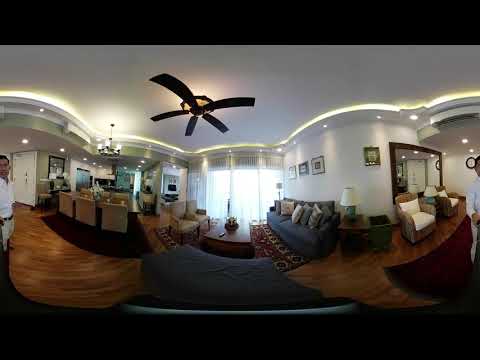This image captures the open interior of a luxurious and spacious house, blending a kitchen on the left with a living or family room on the right. The white walls and ceiling create a bright and airy environment, accentuated by a ceiling fan positioned centrally, which is turned off. A lens with a distinctive distortion effect has been used, bending spatial lines and producing a unique, aesthetically pleasing curvature in the photograph. On the far left, you can see the person taking the photo, dressed in a white shirt and pants, while on the right, another portion of a potential second person is partially visible—though due to the lens distortion, it might be the same individual.

The living room area is furnished with an array of high-quality pieces, including couches, seats, tables, and coffee tables, thoughtfully arranged to create a balanced and inviting space. Along the right side, there's an alcove featuring a mirror, and the room is illuminated by bright sunlight streaming through a large, possibly sliding, porch door—suggesting high-end construction and materials. The floor is streaked with elegant paneling, adding to the room's sophisticated character. Overall, the mix of blues, browns, and whites in the decor contributes to the stylish and well-coordinated ambience, making it a dream space one would love to live in.